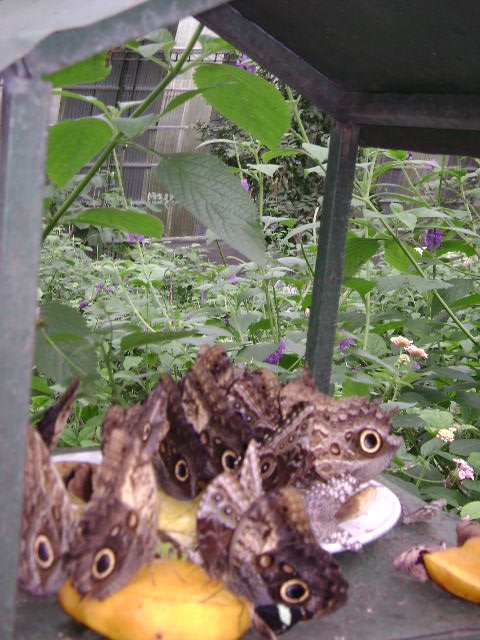In a lush, verdant garden, an intricately arranged enclosure takes center stage, teeming with a fluttering spectacle of owl butterflies. These extraordinary creatures, recognized by the eye-like patterns on their brown, spotted wings, are seen resting with their wings outstretched. This natural camouflage deceives potential predators, making them blend seamlessly with their surroundings. Nestled within the enclosure are pieces of fruit, likely mango or cantaloupe, skillfully laid out to attract these fascinating insects. The fruit-laden scene hosts about half a dozen butterflies, some clustered around a silver platter, while others gravitate towards smaller pieces of fruit, all facing different directions in their gentle repose.

In the background, the environment transitions into a lush, residential area, marked by a fence and an array of plants adorned with purple, white, and yellow flowers. The vegetation, dense and vibrant, hints at a warm, possibly tropical climate, ideal for the thriving flora and the butterflies they attract. This meticulously captured moment in the garden showcases not just the beauty of the butterflies but also the harmonious interplay between nature and its spectators.